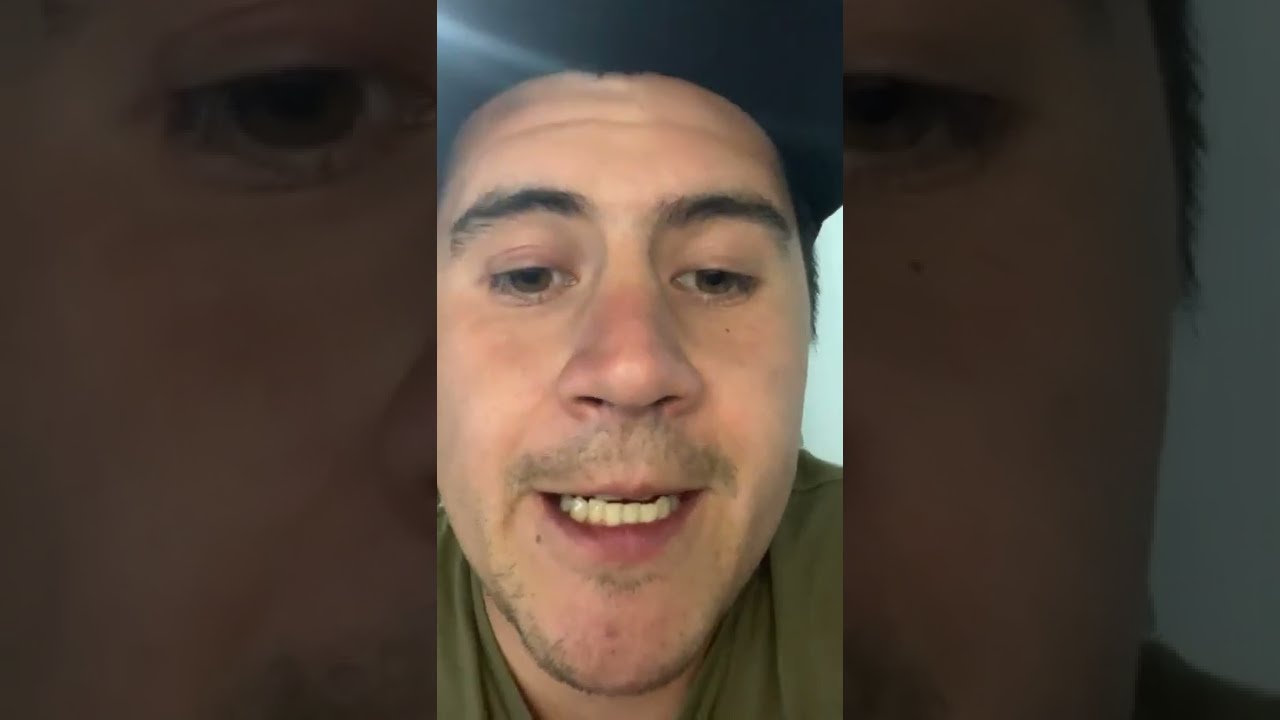The image is divided into three vertical sections, showcasing a close-up of a man's face. The outer sections darken and replicate the image in the middle. The man, appearing to be in his 30s, has light skin with dark stubble, particularly a light mustache and spots of facial hair on his chin. He has striking bushy black eyebrows and expressive greenish-brown eyes that are half-closed, glancing slightly downward. His mouth is slightly open, revealing his lower teeth. His lips are a deep red shade. He sports a baseball cap, partially obscuring his forehead, and wears a baggy olive green t-shirt. In the background, a faint light blue wall is visible. The photograph captures the nuanced, textured elements of his face and attire, creating a layered, intimate portrayal.